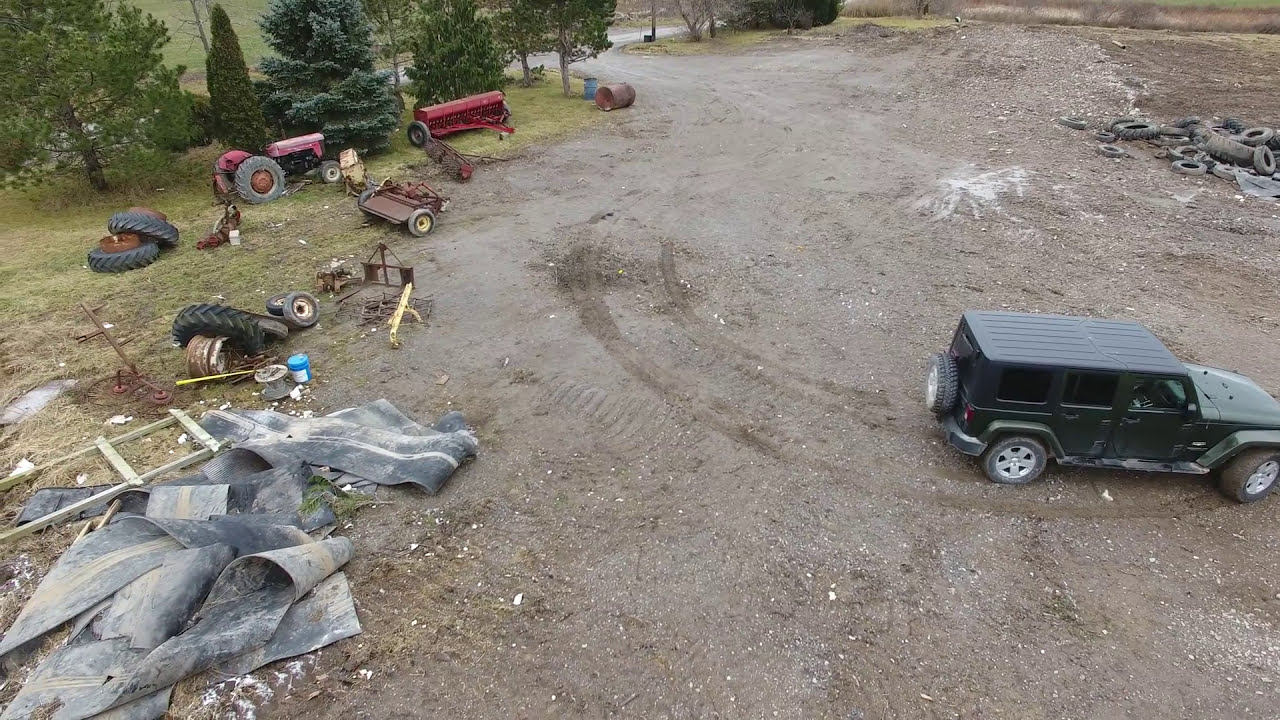The image depicts an outdoor area, likely a dirt road, driveway, or dump site, characterized by a mix of bare earth and gravel, particularly prominent along the right side. A green, four-door Jeep Wrangler-type vehicle is parked near the bottom right, pointing to the right. Above it, in the top right corner, there is a pile of discarded tires. The top left corner showcases a variety of lush, green trees. The left side of the image is cluttered with various discarded items, including large tires, pieces of farm equipment, wheels, and strips of black fabric or possibly tar paper. Among the scattered items, there also appears to be a lattice for climbing plants. The foreground of this left side prominently features a grayish mass of material, which could be plastic or rubber sheets. Overall, the scene is dominated by discarded objects and debris against a backdrop of natural greenery and bare earth.